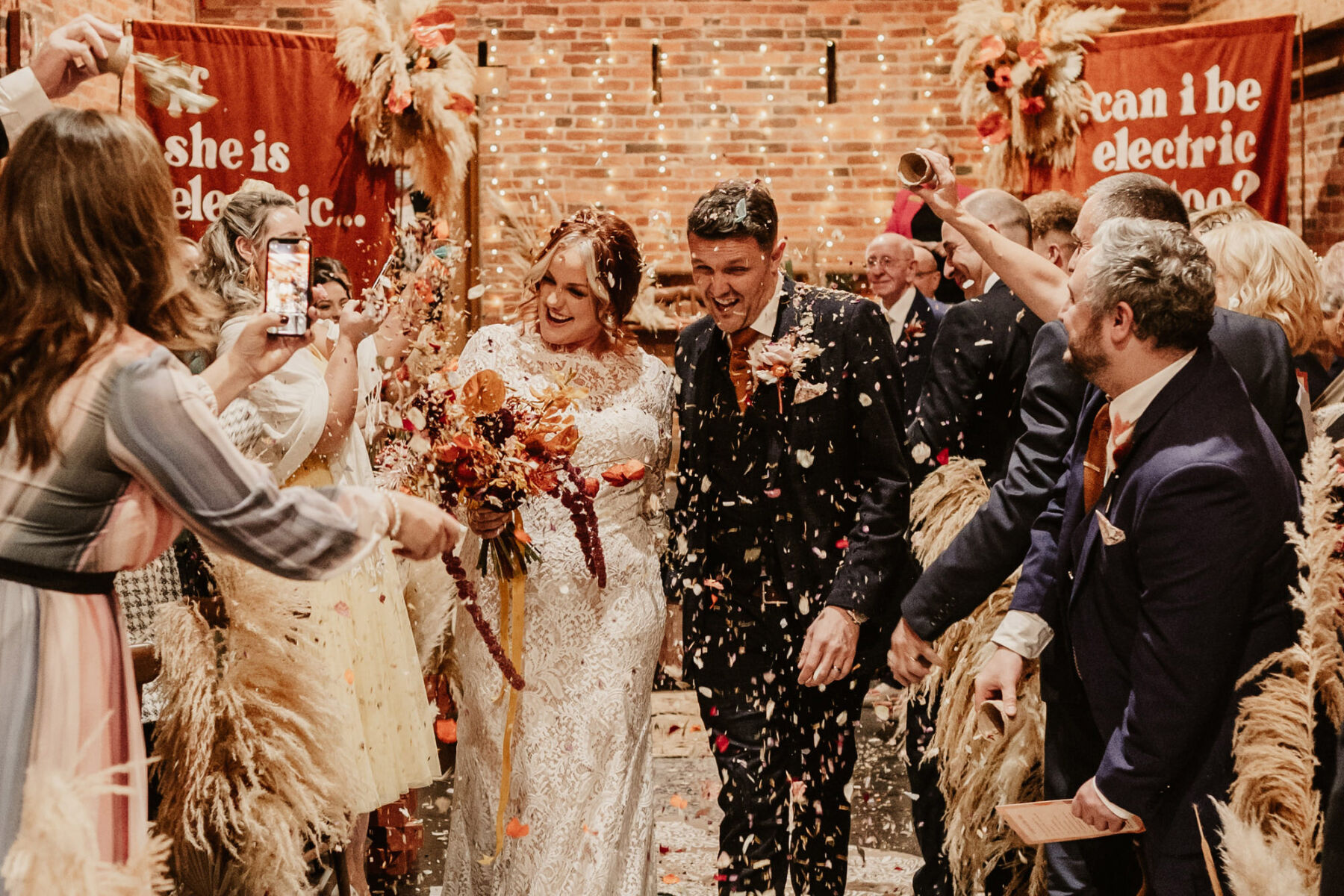In the wedding photograph, the newly married bride and groom are joyously walking down a narrow, confetti-filled aisle, lit warmly by fairy lights strung against a brick wall. The bride, radiant in her flowing white gown, holds a bouquet of autumn-colored flowers, while the groom, beaming in his suit and reddish-orange tie, sports a boutonniere on his chest pocket. On either side of the aisle, a large group of excited guests, predominantly women, are showering the couple with confetti and capturing the moment with their smartphones. Prominent in the scene are two red banners with white text, likely referencing the band Oasis, reading "She is electric" and "Can I be electric too?" A tall woman stands in the foreground as the couple approaches her, moving through the bustling, celebratory crowd.